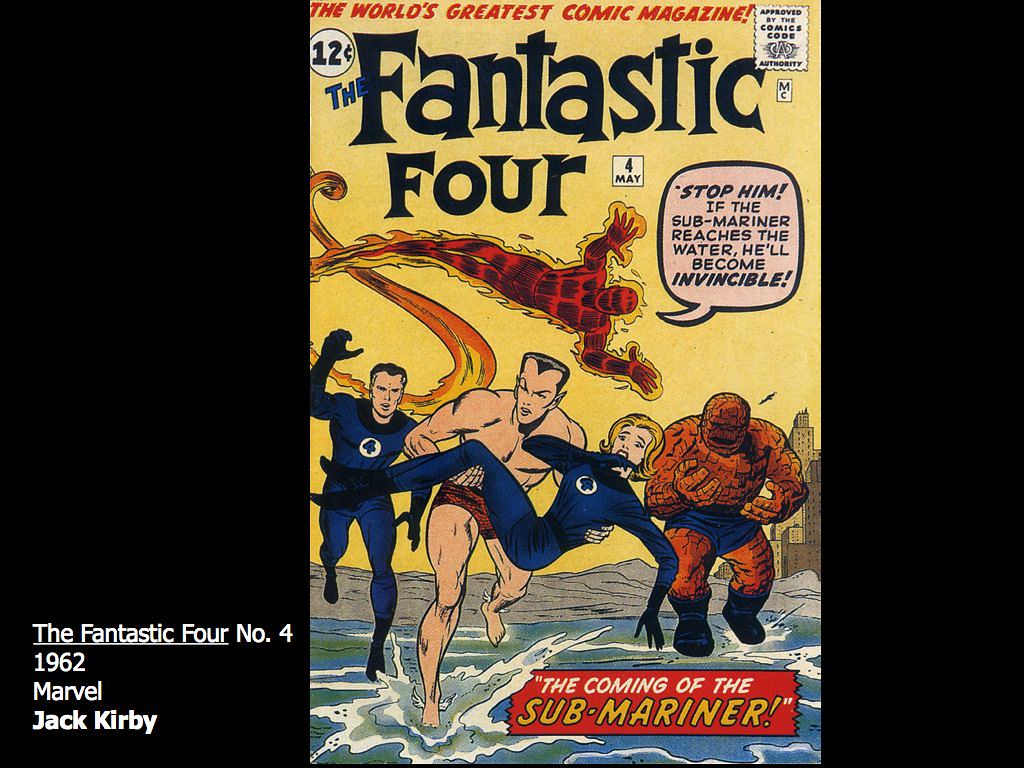The image depicts a comic book cover titled "The World's Greatest Comic Magazine" in red at the top, set against a predominantly yellowish sky. Near the top, a dialogue bubble from a superhero flying across the sky in a reddish-orange form reads, "To Fantastic Four: stop him! If the Submariner reaches the water, he'll become invisible!" Below, the scene features five distinct characters. The superhero on fire is flying, and there is also a rock-like man wearing blue trunks and boots. Another figure in green scaly trunks with pointy ears and small wings on his feet is carrying a woman in a blue suit emblazoned with a '4', heading towards the water. A second man, also in a blue suit with a '4' on his chest, chases after the kidnapper. At the bottom of the cover, text announces "The Coming of the Submariner," and in the bottom left corner, it reads, "The Fantastic Four, Number Four, 1962 Marvel, Jack Kirby."